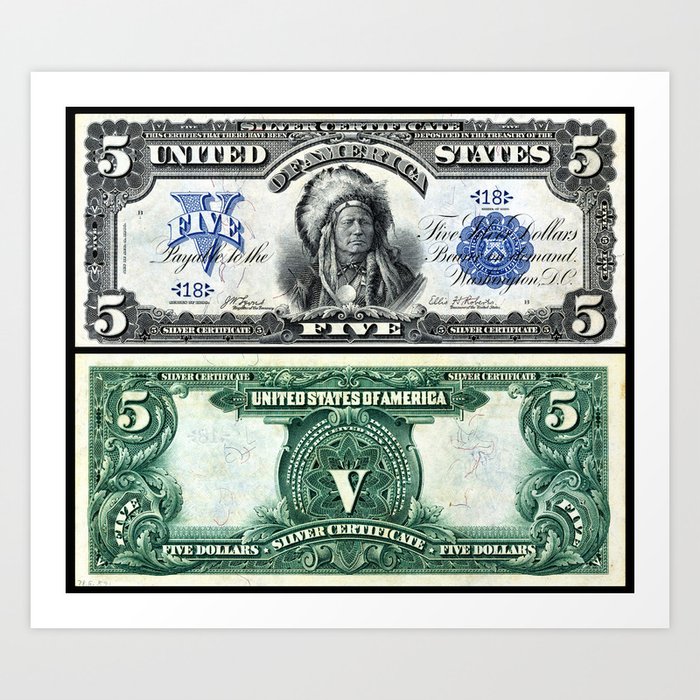The image depicts a white-framed $5 U.S. silver certificate displayed front and back, set against a light blue background. The top half showcases the obverse of the note, primarily rendered in black, gray, and blue ink. At its center is the portrait of a Native American chief, contrasting traditional designs. Four numerical "5s" occupy each corner, with additional blue elements, including a Roman numeral "V" on the left and a blue government seal on the right. The reverse, displayed on the bottom half, is primarily in shades of green, adorned with intricate filigree patterns. The back prominently features a large "V" in the center and the text "United States of America" at the top, with the denomination "$5" repeated in the corners. The note is styled similarly to modern currency, maintaining a familiar rectangular shape, but its unique details suggest historical significance.